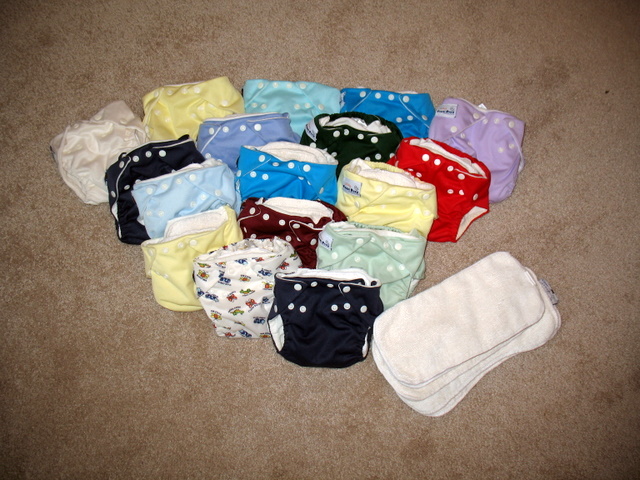This image showcases an array of reusable, washable diapers meticulously arranged on a brown carpet. The diapers are displayed in a staggered configuration, starting with one in the forefront and gradually increasing to five in the background. The diapers feature a variety of vibrant colors and patterns, including solid hues, polka dots, and playful prints. On the top row, from right to left, the colors progress from purple, blue, teal, yellow, to cream white, some adorned with round white circles. The second row includes red, black, light blue, another black with white circles, followed by yellow, blue, and teal with additional white circles. The third row consists of teal, dark red, and yellow, while the bottom has two black diapers and one white diaper with red, orange, and blue designs. To the bottom right of the image, a stack of short, white washcloths or cloth pads, used as inserts for the diapers, is visible. The diapers are equipped with adjustable snaps and elastic leg openings to fit various sizes, showcasing both functionality and colorful diversity.